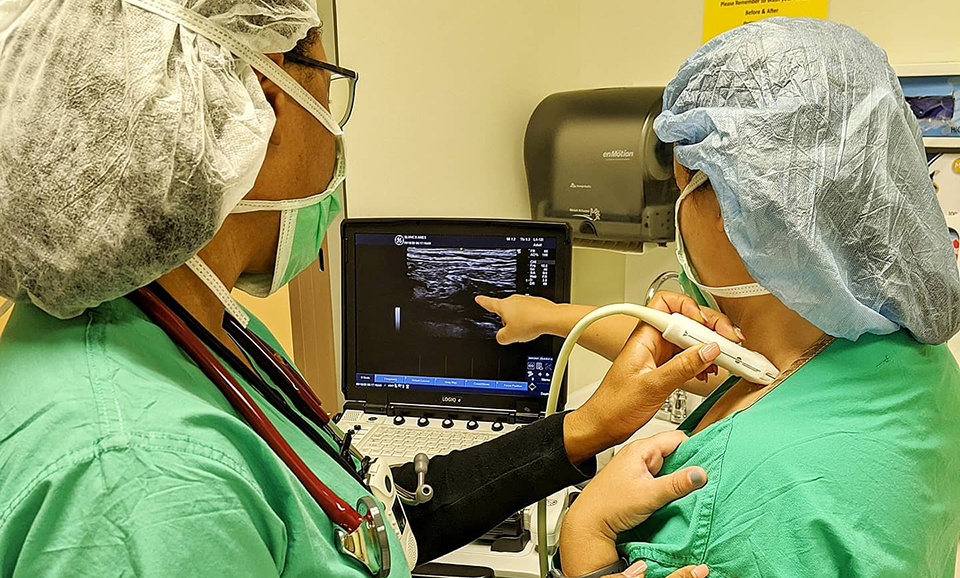This image depicts two medical professionals, likely nurses or doctors, stationed in a clinical environment. Both individuals are clad in green scrubs and are adorned with face masks and hairnets. The person on the left, who is darker-skinned and bespectacled, also wears a stethoscope and what appears to be a pulse oximeter around her neck. She is layered with a black long-sleeve shirt underneath her scrub top and is holding an ultrasound wand in her left hand, positioning it just below the neckline of the second person. This second individual, with lighter skin, is slightly adjusting her scrub neckline with her left hand, while her right finger points towards an ultrasound screen that displays the ongoing examination. Both are intently focused on this screen. In the background, a paper towel dispenser and a partial view of a door are visible against the clinical office walls.